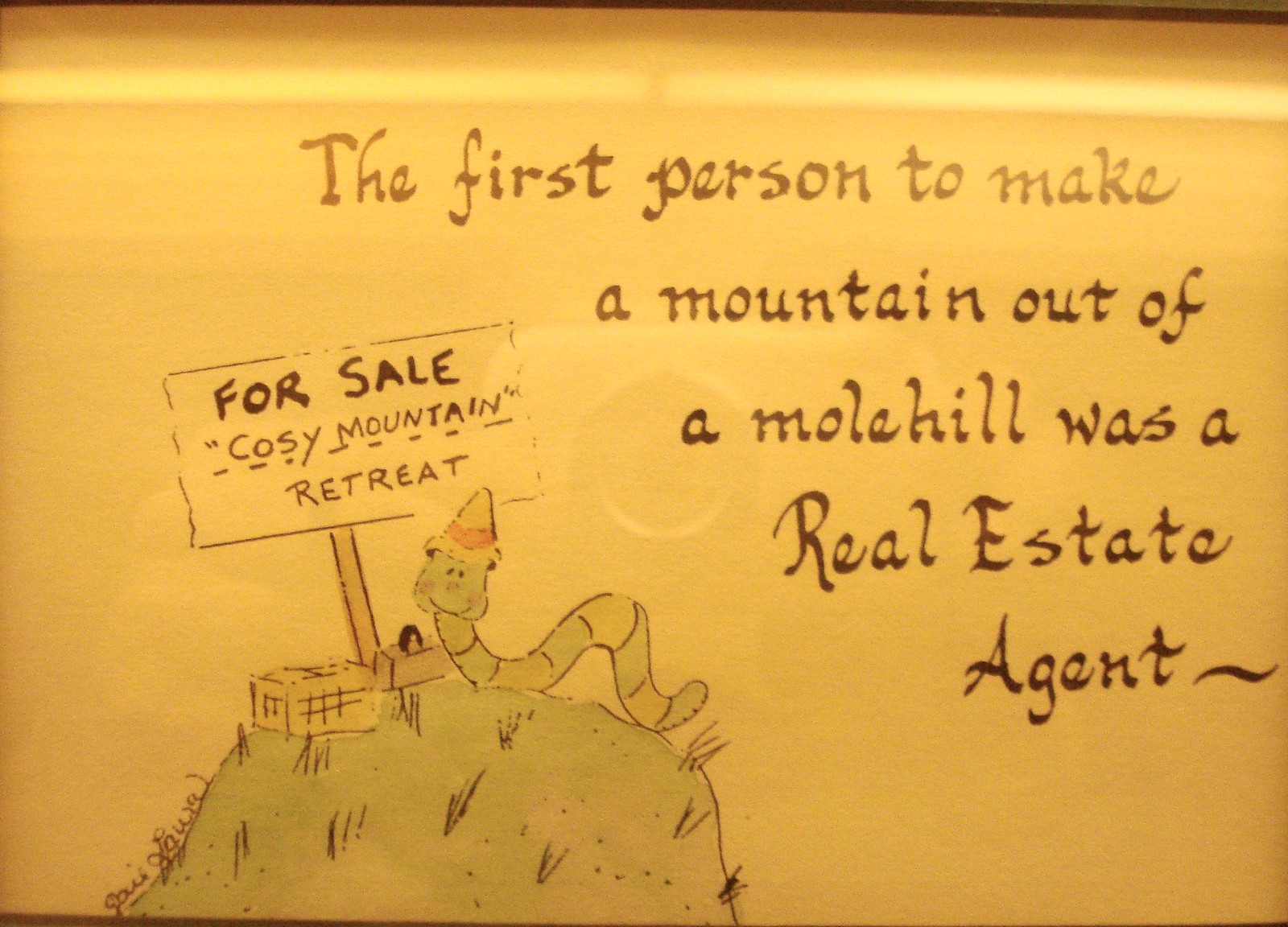The image features a whimsical drawing of a green hill with a grassy texture, under a white background. Atop the hill sits a smiling green worm, distinguished by its triangular red, white, and yellow hat. The scene includes a picnic setup with a lunchbox and a basket beside the worm. A sign emerging from the hill reads "For Sale: Cozy Mountain Retreat." Above and to the right of the scene is text written in black ink that humorously states, "The first person to make a mountain out of a molehill was a real estate agent." This artistic piece, possibly intended as a meme, has a signature by the artist, which appears to be Gail Lawa, although it is somewhat hard to decipher. The photograph of the drawing is tinged with yellow light and seems to be behind glass, resulting in reflections. There is equipment visible in the background, adding to the impression that this is part of a display or advertisement for real estate.